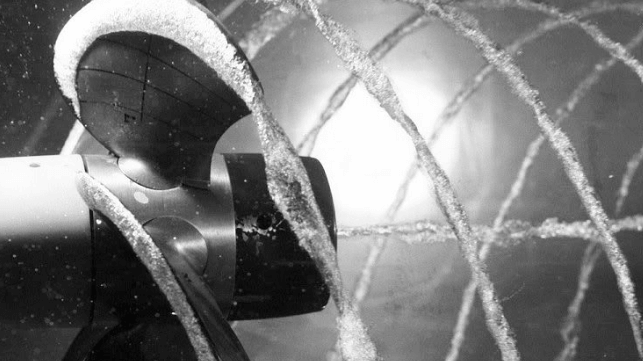This highly zoomed-in black and white image exudes an artsy, abstract feel. Dominated by various shades of gray, it portrays a scene that appears to center around a metallic, machine-like object featuring fan fins on one side. While the object could potentially be part of a sprinkler or fountain system, it's clear that water is an integral element of the scene. Visible water sprinklers and splatters surround the machine, creating swirling patterns and a direct line of water shooting out across the frame. Adding to the intrigue, the background is blurred and features a bright light source, perhaps a big bulb, adding an ethereal glow to the composition. White and gray elements interlace, with some areas taking on a web-like appearance, producing a mystifying and captivating visual experience.